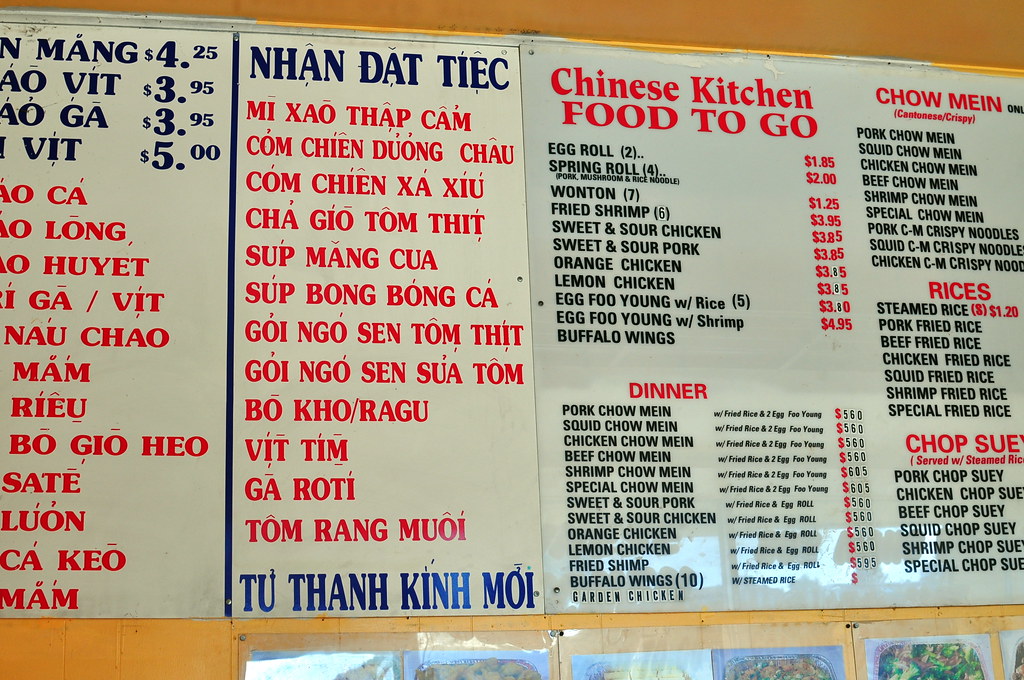This is an image of an extensive menu typically found in a restaurant. The menu is in a landscape orientation and occupies about 90% of the visible area. The menu is divided into three distinct sections. 

On the left, there is a white, portrait-style menu that is partially cut off, showing only halfway. Beside it is another white, portrait-style menu of a similar size; together, these two sections form approximately half of the entire menu's width. The rightmost section is a larger, square-shaped menu that is the size of the two left sections combined. This square menu features a slightly different shade of white, appearing more grayish.

The square menu is headlined with "Chinese Food To Go" in prominent red letters. Below this heading, there are various items listed for sale, categorized under "Appetizers" and "Dinner" also in red text. The right side lists options like chow mein, rice dishes, and chop suey. The left side uses blue lettering for prices, while the food items are listed in red. The names of the food items are written in a foreign language, which is not identifiable or readable by the viewer.

Additionally, below the second portrait menu, there is blue lettering in another foreign language. Underneath this text, the wall is adorned with pictures of food items, serving as visual examples of the dishes available for purchase at the restaurant.